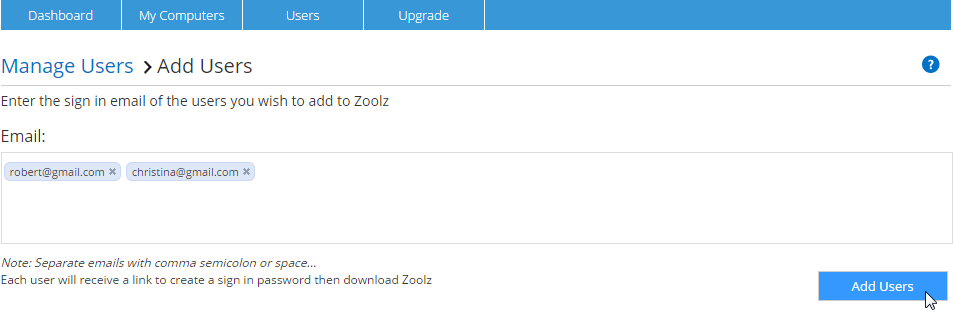The image features a user interface for managing users in a software application named Zootz. At the top, there is a long blue rectangle divided into four sections by small white vertical lines, each labeled in sequence from left to right: "Dashboard," "My Computers," "Users," and "Upgrade." 

Beneath this, in blue text, appear the phrases "Manage Users" followed by a right-pointing arrow, and "Add Users." These are underlined by an extended horizontal line. The next section provides instructions: "Enter the sign-in email of the users you wish to add to Zoots (Z-O-O-T-Z)."

Below the instructions, there is a label reading "Email:" followed by two example email addresses displayed within blue rectangles: "robert@gmail.com" and "christina@gmail.com." 

At the bottom left of the screen, a note instructs, "Separate emails with a comma, semicolon, or space. Each user will receive a link to create a sign-in password, then download Zootz (Z-O-O-L-Z)."

About six inches to the right, there is another blue rectangle with bold lettering inside reading "Add Users."